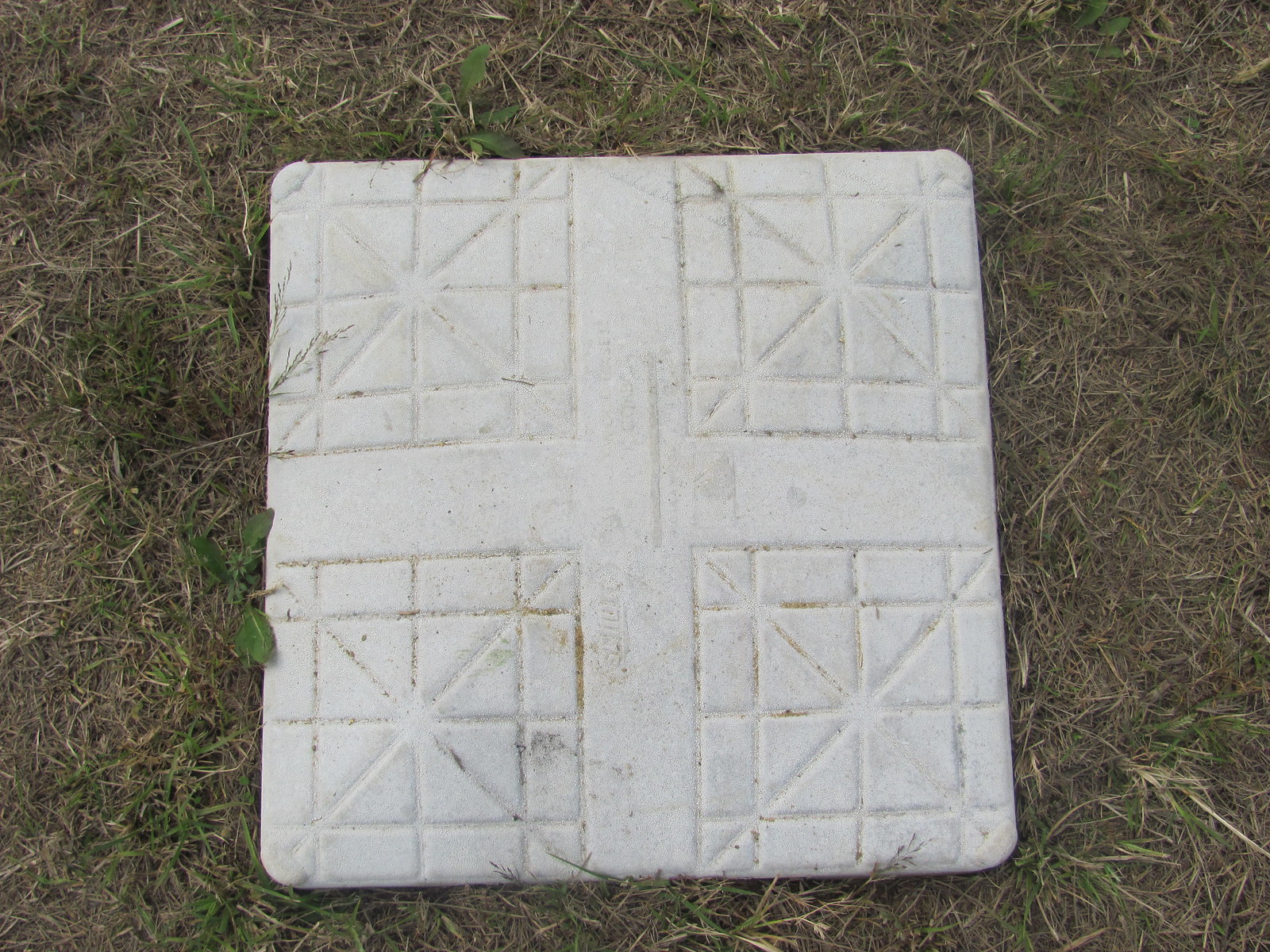This horizontal, rectangular color photograph captures a slightly dirty and well-used baseball base laying on a patch of dry, green grass. The base is a white, slightly rounded square, placed on a slight bias. The center of the base features a prominent cross design created by wide lines. Each quadrant formed by the cross contains identical patterns of small square boxes, each adorned with an intricate star-like design created by radiating lines. Around the sides of these quadrants are additional squares and rectangles, each embellished with a cross or X, maintaining the symmetrical, repetitive pattern across the entire base. The base shows scuffs and marks indicative of frequent use, with a faint, unreadable brand name slightly raised in the lower center portion of the cross.